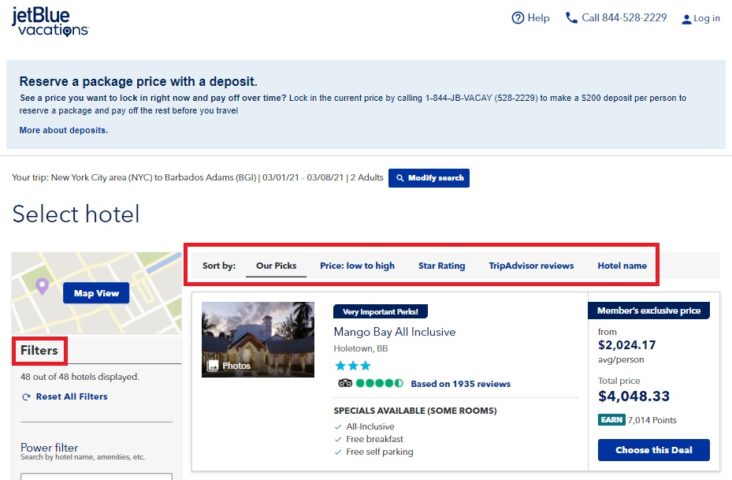**Descriptive Caption:**

The screenshot features the JetBlue Vacations webpage. In the header, "JetBlue Vacations" is prominently displayed on the top left, while on the top right, there are options for assistance, including a help link, a contact number (844-528-2229), and a log-in prompt. Below the header, there is a call-to-action: "Reserve a package price with a deposit. See a price you want to lock in right now and pay off over time." It provides instructions to lock in the current price by calling 1-844-JB-VACAY-528-2229, requiring a $200 deposit per person to secure the package and pay off the rest before travel.

The highlighted trip is from New York City (NYC) to Grantley Adams International Airport (BGI) in Barbados, scheduled from March 1, 2021, to March 8, 2021, for two adults. Options to modify the search, select a hotel, view on a map, and apply filters are available. The Filters section is outlined in red, showing 48 out of 48 hotels displayed with options to reset all filters or use the power filter to search by hotel name and amenities.

To the right, there's a menu bar outlined in red with sorting options by recommended picks, price (low to high), star rating, TripAdvisor reviews, and hotel name. The central photo is of a picturesque hotel silhouetted against a sunset sky. It features details about Mango Bay, an all-inclusive hotel in Holetown, Barbados, rated 3 stars and with a TripAdvisor rating of 4.5 based on 1,935 reviews. Special offers are noted, including some rooms being all-inclusive, free breakfast, and free self-parking. The members' exclusive price starts from $2,024.17 per person, with a total package cost of $4,048.33 and an opportunity to earn 7,014 points. The caption concludes with an invitation to "Choose this deal."